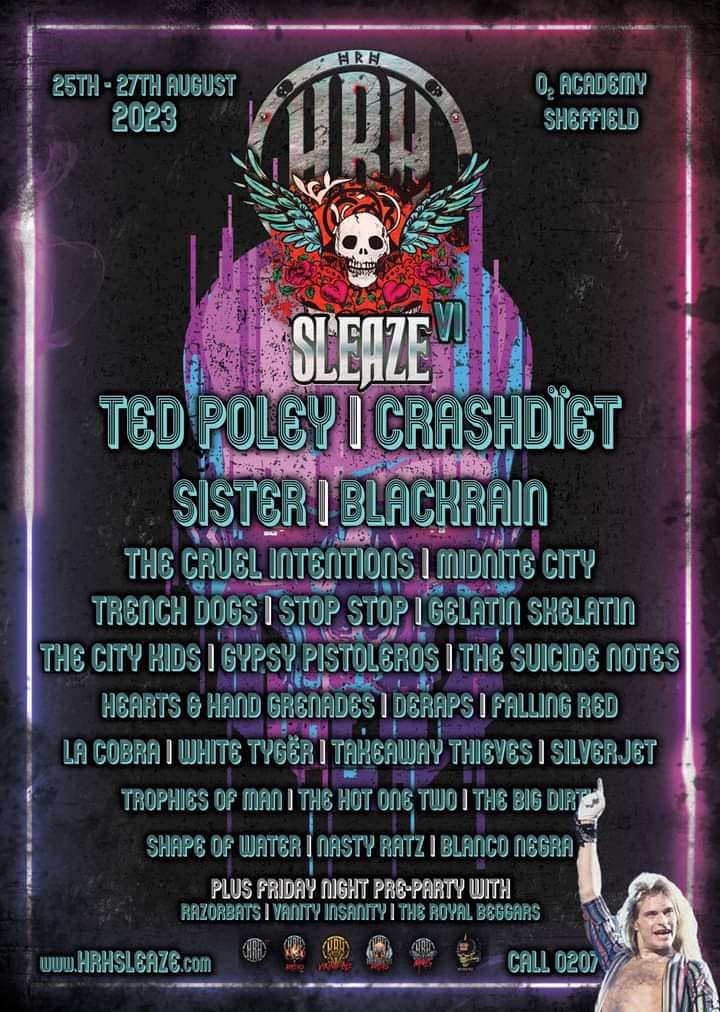The poster is an advertisement for a rock concert taking place from August 25th to 27th, 2023, at the O2 Academy in Sheffield, organized by HRH (Hero Academy Sheffield). Dominated by a dark theme with neon purple and teal accents, the poster prominently features a striking white skull with wings or olive branches on either side, set against a backdrop of red and purple flowers. The main text highlights "Sleaze VI" in the center, indicating the headlining band Sleaze. Below this, numerous bands are listed in teal and green fonts including The Cruel Intentions, Midnight City, Ted Pauly, Crash Site, Sister, Black Rain, Trench Dogs, Stop Stop, Gelatin Shelatin, The City Kids, Suicide Notes, Gypsy Pistoleros, Hearts and Hand Grenades, D-Wraps, Falling Red, LA Cobra, White Tiger, Takeaway Thieves, Silver Jet, Trophies of Man, The Hot One Two, The Big Dirty, Shape of Water, Nasty Ratz, and Blanco Negra. There is also a note about a Friday night pre-party featuring Razor Brats, Vanity Insane, and The Royal Beggars. The bottom left corner includes a partially obscured website, "HRHSleaze.com". The bottom right features a contact number alongside an image of a Caucasian man with long blonde hair, wearing a strapped blue and pink shirt and a black bracelet, raising his hand. Overall, the poster conveys a lively and vibrant promotional piece for a massive multi-day rock event.